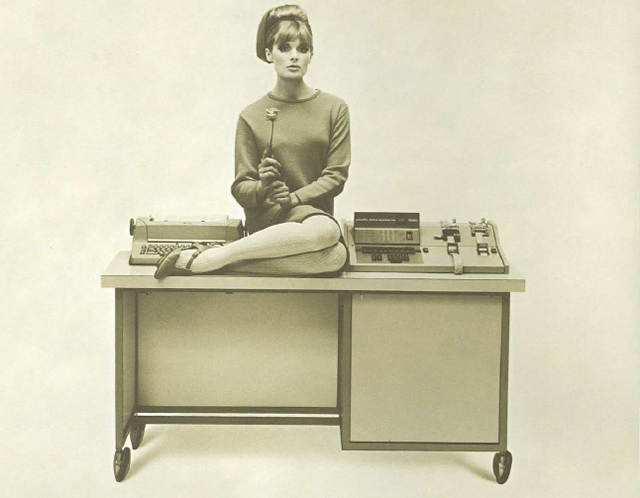This image is a detailed vintage photograph from the 1960s, adopting a sepia tone. At its center is a young Caucasian woman, likely in her 20s, possibly a model or actress, embodying a mod culture style. Her hair is pulled back in a ponytail with a puffy effect, characteristic of the era. She is wearing a long-sleeved mini-dress with a circle neck, resting on top of a desk that features a light-colored wooden top and dark gray metal frame with caster wheels. The desk includes a cubby on the bottom left, designed for an office setting. 

The woman, who has her legs bent and folded on the desk in front of her, is holding a rose with both hands, adding a touch of romanticism to the scene. To her left is an electric typewriter, a prominent office fixture of the time, while to her right is an old computer-like device featuring keys and a small LED screen displaying text, possibly used for ticker tape, indicative of stock market operations. Her poised and enigmatic expression, coupled with the vintage office equipment, suggests this might be an old advertisement, rich in nostalgic charm.